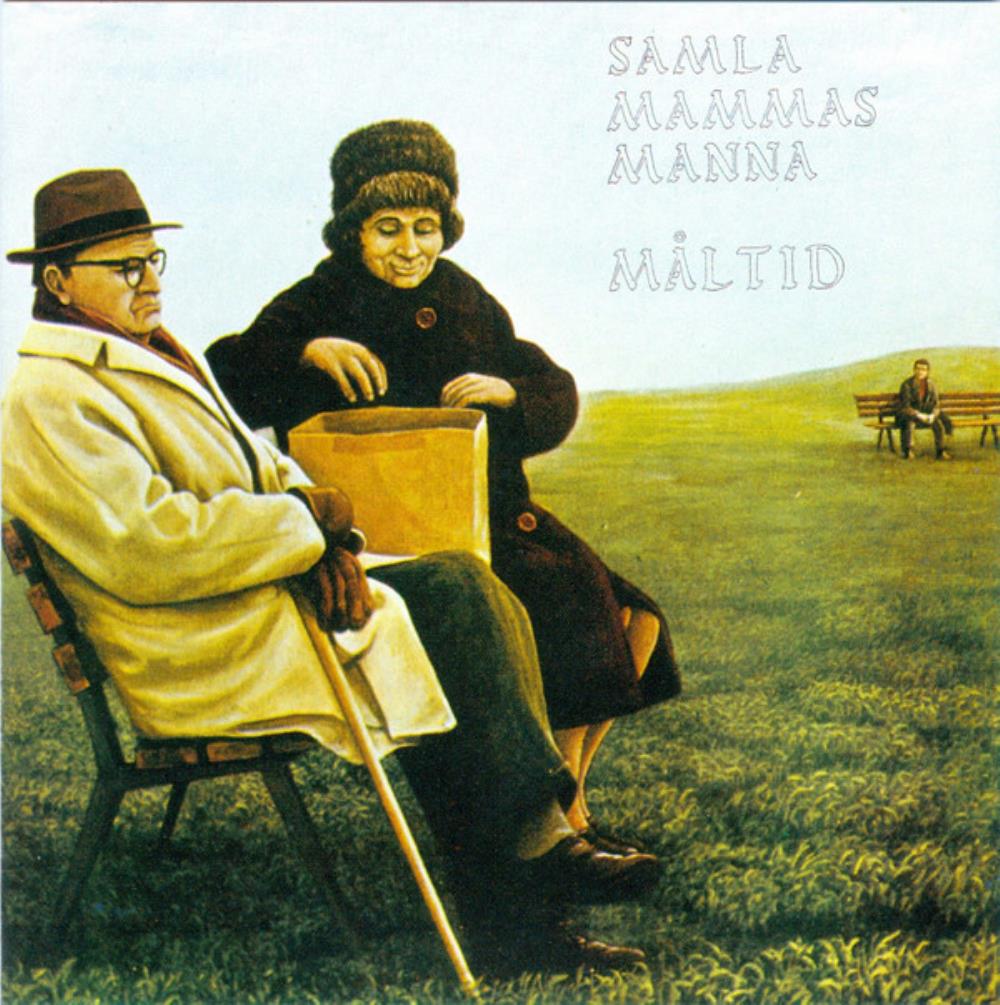The image is a hyper-realistic drawing, possibly a painting or an advertisement, depicting an outdoor scene with a pale blue sky and a vast green field. In the foreground, an older gentleman and an older woman are seated on a wooden bench that is oriented to the side. The gentleman, who has a scowl on his face, is wearing a distinctive ensemble comprising a white overcoat, dark pants, and dark brown shoes. He accessorizes with leather gloves, a scarf, eyeglasses, a cane leaning against him, and a distinctive top hat. His legs are crossed, and his arms are folded in his lap as he looks down at the ground. Beside him, the older woman, with a pleasant expression and short, curled under dark hair, is dressed in a thick, dark brown coat with large light brown buttons and a brown fur hat. She appears to be reaching into a folded paper sack placed between her and the gentleman. In the background, another bench recedes into the distance, where a younger individual dressed in dark clothing sits, leaning forward on their knees, observing the older pair. The scene is accentuated with foreign text in the top right corner that reads "Samla, Mamas, Mana, Maltid."